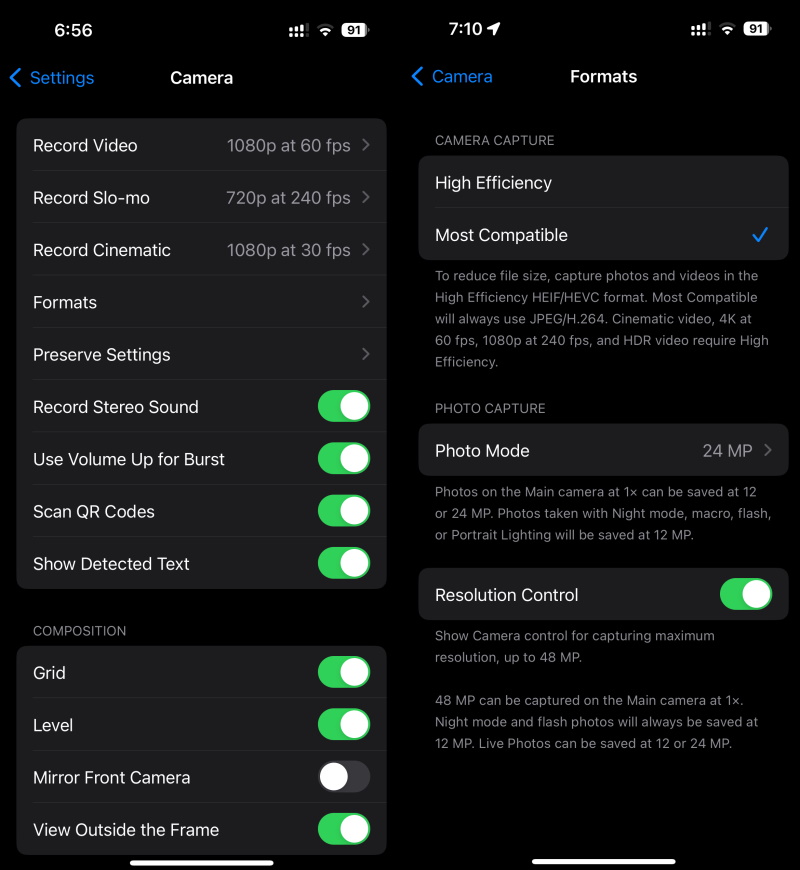This is a detailed screenshot of a settings page, presented as two screenshots placed side-by-side, showcasing the Camera settings in dark mode. On the top left of the left screenshot, a blue "Settings" title is displayed with a blue back arrow to its left. Both screenshots feature a dark background with light text, and various options are highlighted against dark grey sections.

The first section, titled "Camera," lists multiple settings including Record Video, Record Slow-Mo, Record Cinematic Formats, Preserve Settings, Record Stereo Sound, Use Volume Up for Burst, Scan QR Codes, and Show Detected Text. The latter four options have green toggle buttons on the right side, indicating they are enabled. 

Further down, the settings continue with "Composition" options, which include Grid, Level, Mirror Front Camera, and View Outside the Frame. These intricately presented settings offer a comprehensive overview of the camera customization options available in the app.